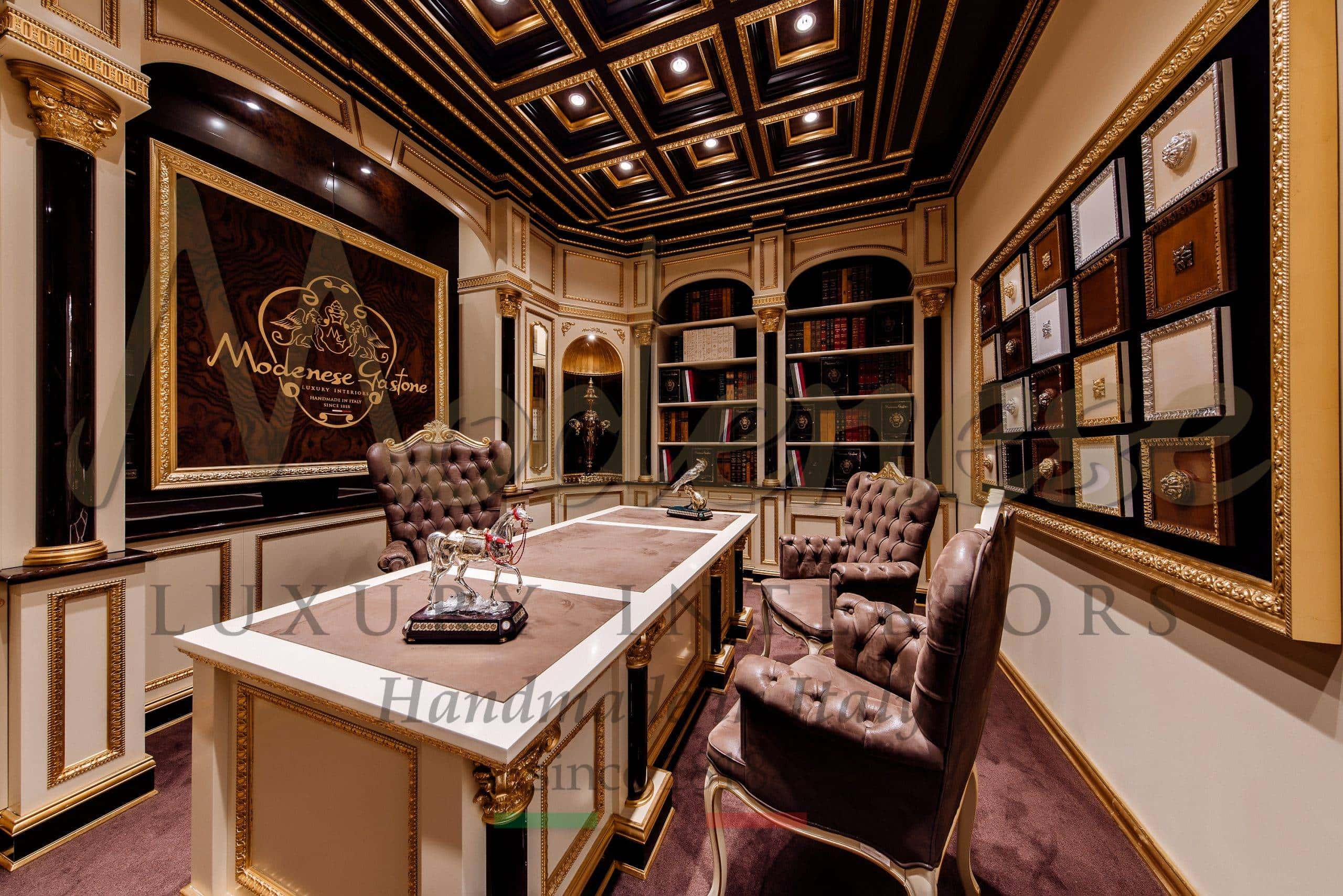The photograph captures the interior of an opulently designed office, showcasing an exquisite blend of earthy tones and luxurious décor. Dominating the room is a long, rectangular desk complemented by two plush, brown leather armchairs designated for clients, positioned in front. Behind the desk, angled towards the viewer, is a sumptuous purplish-brown leather swivel chair for the office's occupant. The back wall features extensive bookshelves filled with numerous volumes, lending a scholarly ambiance to the space.

The office boasts a dark paneled ceiling adorned with recessed lights set inside gold-accented squares, adding an element of grandeur. The walls are predominantly white with gold trims, harmonizing with the room's brownish-reddish carpet. On the right side, an art piece in a large gold frame adds to the aesthetic richness. Additionally, the desk is decorated with a silver horse statue and a bird statue perched on a branch, enhancing the luxurious atmosphere.

A significant focal point is a large gold-outlined sign behind the desk that reads "MODENESE GASTONE," with "luxury interiors, handmade in Italy" inscribed underneath, affirming the space's elite origins. The overall decor, featuring various gold and black details, underscores the sophisticated elegance and high-quality craftsmanship of this luxurious office.